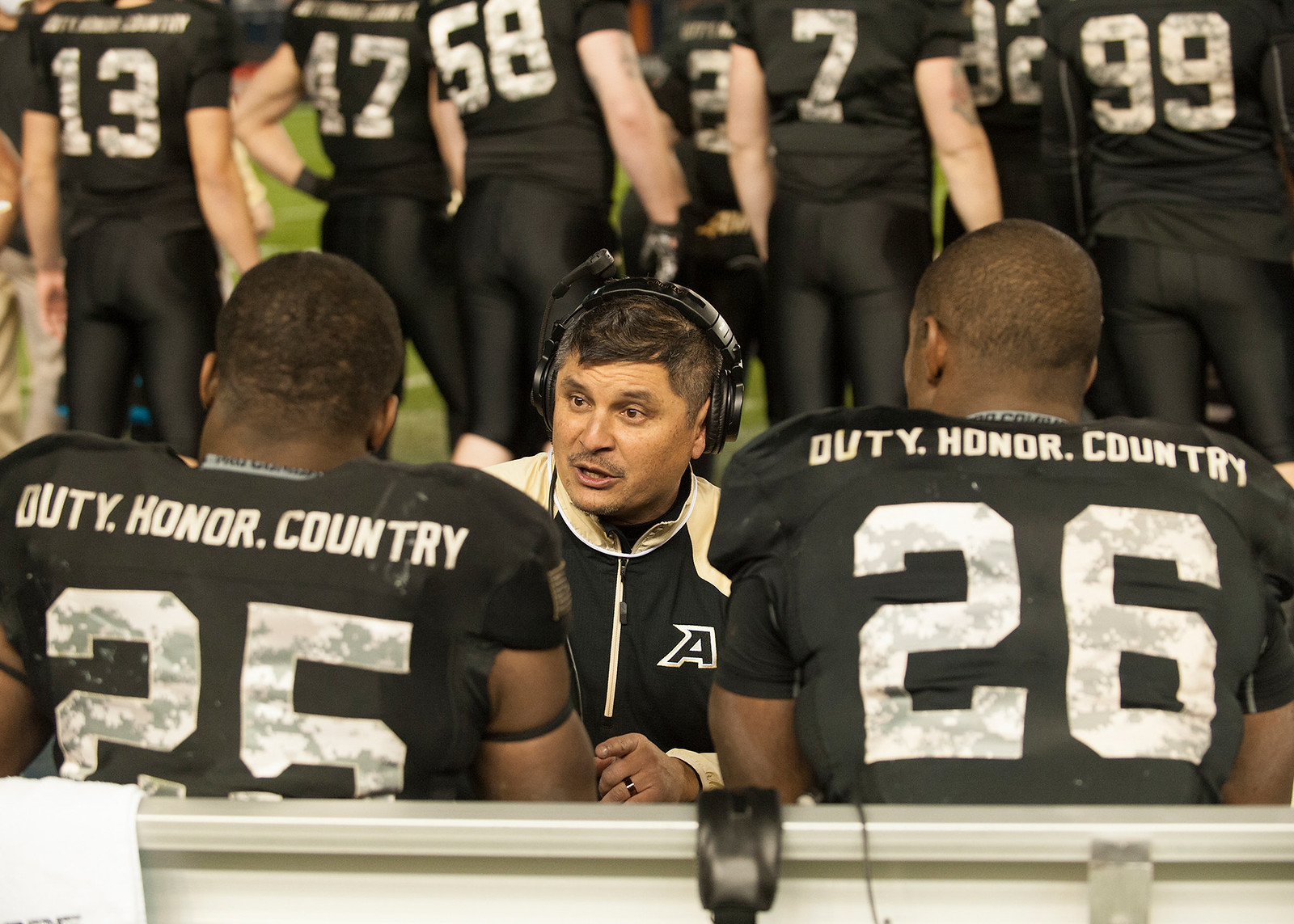In the image, an outdoor football game unfolds on a lush green field with white lines marking the play area. At the forefront, a coach, dressed in a black and white jogging suit adorned with a letter "A," intently engages with two players seated on a silver bench. He wears a black headset and leans towards the players, possibly discussing strategy. The players, clad in black jerseys with the inscriptions "Duty, Honor, Country" on their backs, are number 25 and number 26. Surrounding them, a larger group of teammates can be observed, all similarly dressed in black jerseys and pants with white lettering. Visible jersey numbers in the background include 13, 47, 58, 7, 99, and some partially obscured ones. To the left, partially out of focus, stands an official in a black shirt and chino pants, his bracelet catching the light. Additionally, the bench scene includes a white towel and another set of black headphones, adding to the coaching setup. The overall scene is a dynamic blend of focused preparation and team spirit, set against the backdrop of a vibrant football field.